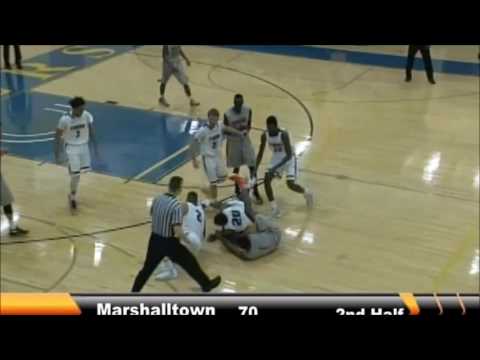This image is a screenshot from a television broadcast of a basketball game. The bottom and top sixths of the image are black, framing a scene on a light tan basketball court highlighted by a blue painted area near the key. In the foreground, a referee in a standard uniform stands observing a scuffle, likely for a loose ball, involving two or three players lying on the floor. One of these players, wearing a white jersey with a number that appears to start with a "2," is from the team Marshalltown, which is leading with 70 points in the second half, as displayed on an orange score banner. Two referees, identifiable only by their black pants, are visible in the background, along with other players who are both engaging with and watching the commotion. The picture does not show the crowd, scoreboard, or hoop, focusing instead on this tense moment on the court.